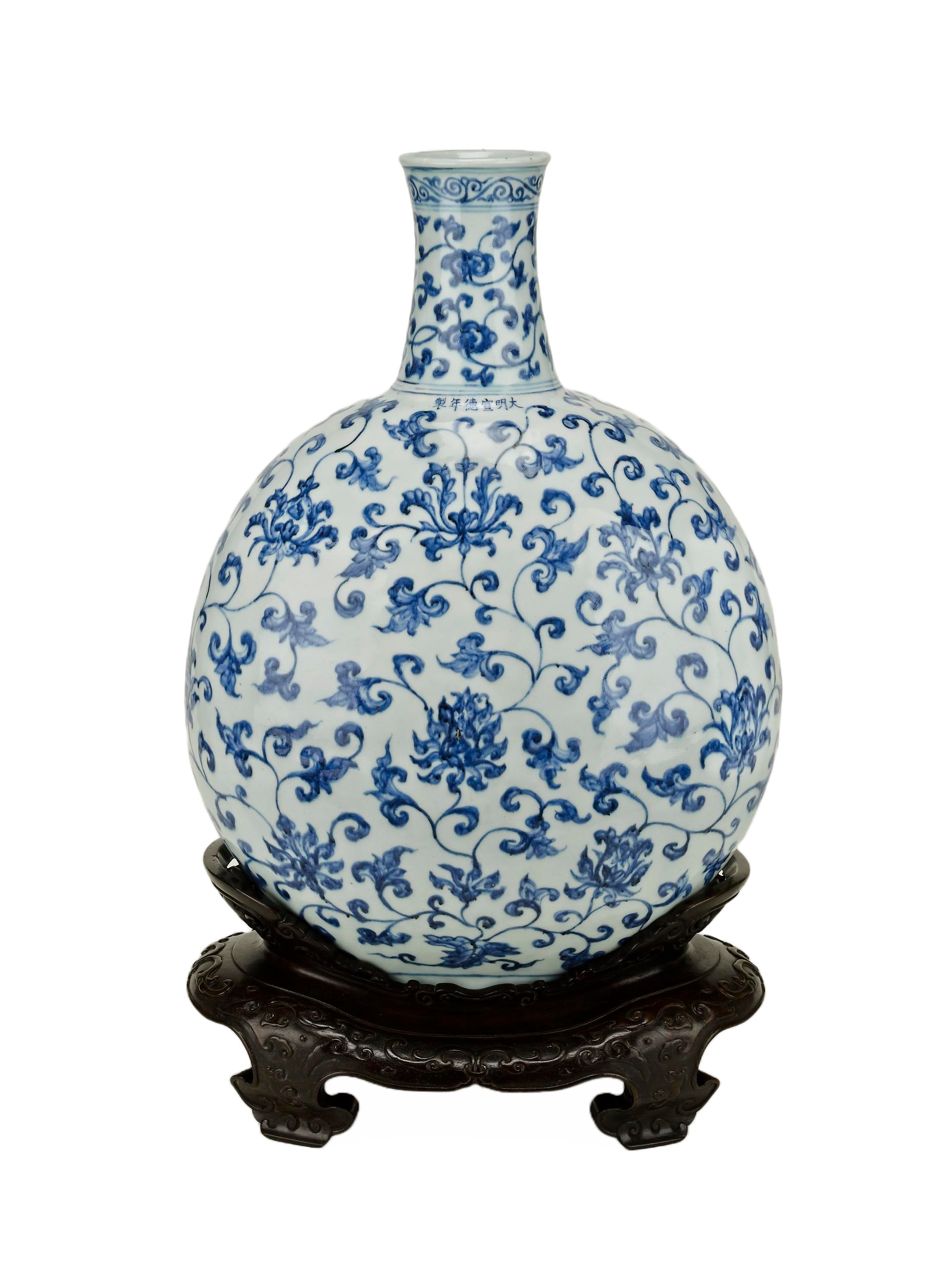This image features an intricately designed oriental ceramic vase, prominently displayed on a decorative stand against a solid white background. The vase itself is predominantly white, shaped as a perfect sphere at its base, culminating in a narrow cylindrical spout at the top. Adorning the vase is a detailed floral pattern in blue, which includes swirling vines, leaves, and variously shaped flowers that appear randomly distributed across the surface. Near the spout, there are Chinese characters inscribed in blue. The vase is elegantly cradled by a black or dark brown pedestal stand, which has an irregular circular shape and short legs that lend a delicate elevation to the display piece. This kind of presentation suggests it might be an artifact for sale or part of a detailed exposition on a specialized website.